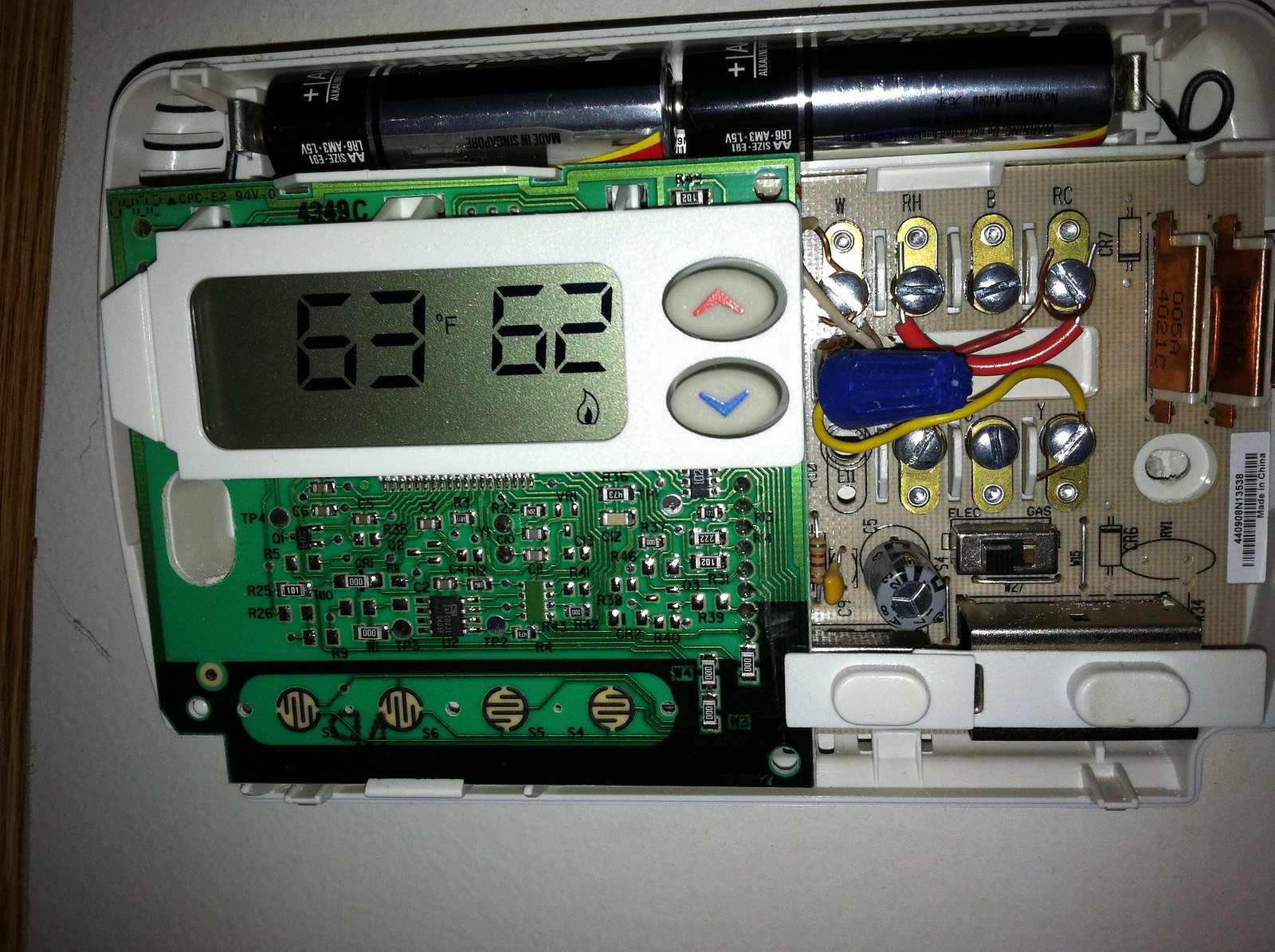This photograph captures a close-up view of a large thermostat mounted on a white slate wall. The wall, adorned with a strip of wood paneling stretching diagonally from the top left to the bottom left corner, provides a contrasting backdrop against the sleek and functional appearance of the thermostat. 

Central to the image is the thermostat itself, featuring a prominent screen on the left side displaying a light green background with readings of 63°F and 62°F, accompanied by a small water drop icon beneath these numbers. Flanking the screen on the right are two vertically aligned buttons; the upper button sports a red arrow pointing up, and the lower button showcases a blue arrow pointing down, presumably for adjusting the temperature settings.

The upper section of the thermostat is distinguished by two black tubes positioned side by side, hinting at its sophisticated design. Below the screen, a glimpse into the inner workings reveals intricate green circuitry interspersed with silver components. Various colorful wires, predominantly yellow and red, are visibly connected, suggesting the complexity and precision of the device. 

Overall, the image meticulously details the appearance and components of the thermostat against the minimalistic aesthetic of the wall, emphasizing the blend of technology and design.